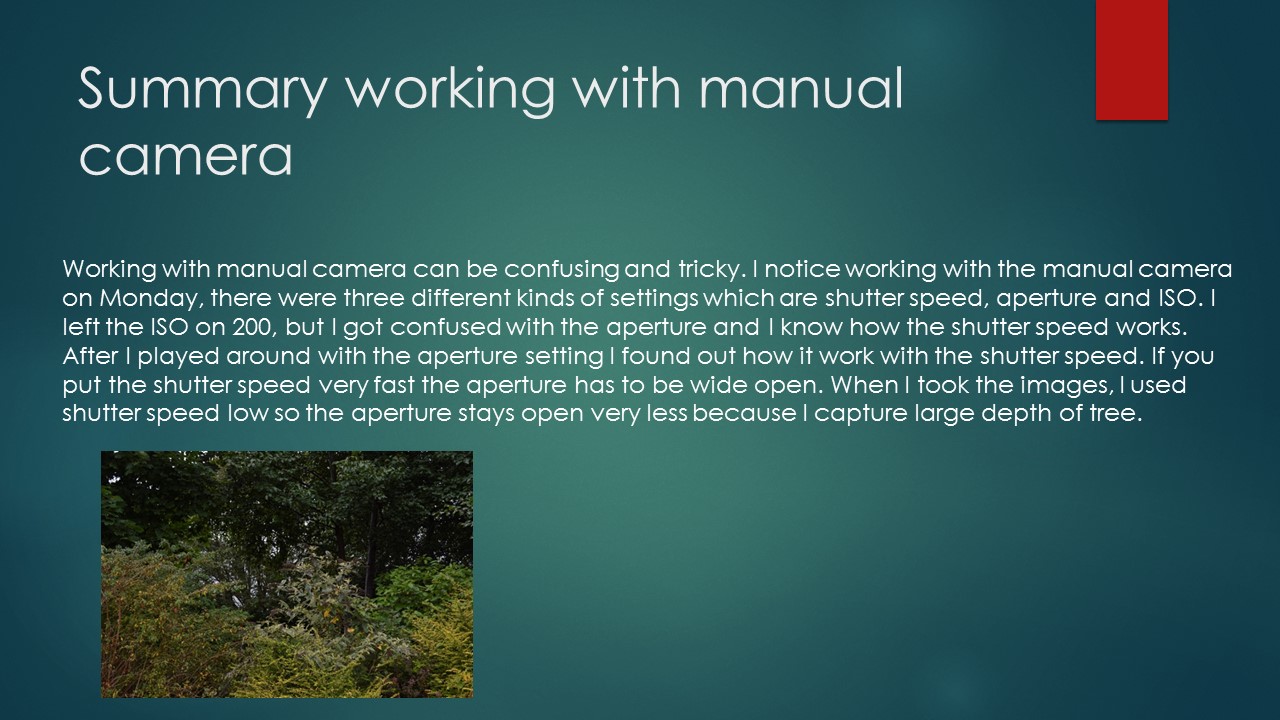The image is a widescreen, high-definition graphic with a dark green gradient background transitioning to a lighter teal glow at the center, and a dark teal at the edges. In the upper left corner, there is a title in white text that reads "Summary Working with Manual Camera." Below the title, there’s a smaller text paragraph beginning with "Working with manual camera can be confusing and tricky." To the right, there is a red ribbon-like bookmark symbol adding a touch of contrast. The paragraph elaborates on various settings of a manual camera, such as shutter speed, aperture, and ISO, describing how these settings interact with each other. The explanation mentions personal experiences, like leaving the ISO at 200, being initially confused by the aperture, and explaining how different shutter speeds impact the aperture for capturing images with large depth of field. Positioned in the bottom left corner is a nature photograph of lush green bushes, exemplifying the manual camera settings discussed in the paragraph. This composition combines textual detail with a visual example, providing a comprehensive guide on operating a manual camera.